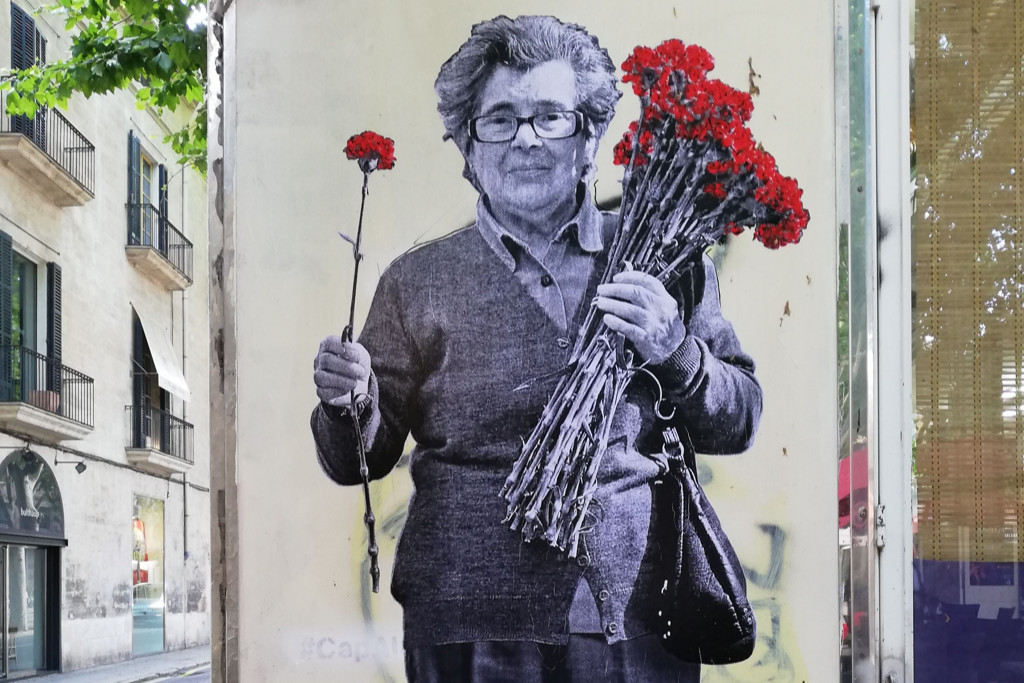This intricate composite image appears to be a carefully crafted collage or photorealistic mural displayed on the side of a building, capturing an essence of vintage charm. Dominating the center is a grainy, black-and-white portrait of an elderly woman, evoking the warmth and gentleness of a grandmother. She wears dark glasses and a cardigan that clings snugly over a collared blouse, revealing a silhouette marked by age. Her naturally gray, short hair contrasts with the neutral tones of her attire. 

The woman is depicted holding a strikingly colorful bouquet in her left hand, a vivid punch of red against the monochrome backdrop. Stalks of roses cascade from her grip, their blooms clustering at the top. In her right hand, she presents a single, equally vibrant, red rose, adding a poignant focal point to her serene, viewer-directed gaze.

Framing her on either side, the image includes snippets of an old suburban environment. To the left, narrow black iron balconies grace the exterior of adjacent buildings, and a leafy tree peeks in from the top left corner, basking in sunlight. On the right, the hint of bamboo behind glass adds an unexpected element of modernity against the otherwise nostalgic scene. The absence of other people and the daytime setting enhance the tranquility and contemplative air of this evocative mural.